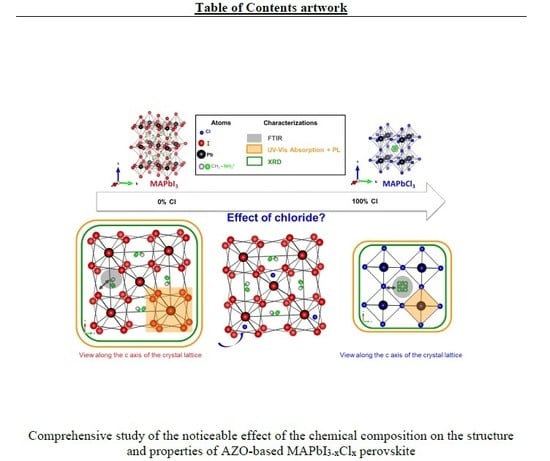The image depicts a detailed scientific diagram titled "Table of Contents Artwork" at the top, suggesting it is from a textbook or scientific paper. The central theme is the "Effect of Chloride," which is visually represented across various diagrams. These diagrams include geometric squares and colored dots (red, blue, and gray) connected by lines, illustrating molecule structures under different chloride conditions, ranging from 0% chloride to 100% chloride. A long arrow highlights this gradient. A key explains the symbols and colors. Beneath the diagrams, a detailed caption reads, "Comprehensive Study of the Noticeable Effect of the Chemical Composition on the Structure and Properties of Azo-Based MAPB I3-X CLX Pervoskite," indicating the scientific focus of the study.